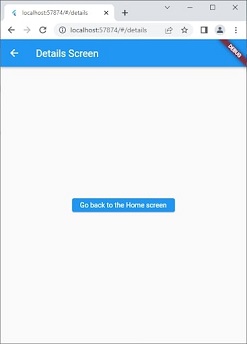A computer screen displays a minimalistic webpage described as a 'detail screen.' Over the right side of the page, there is a maroon diagonal banner. To access this 'detail screen,' users must click on an arrow located underneath the search bar on the left-hand side. Doing so leads to a blank page with a single element: a blue rectangle in the center that reads 'Go Back to the Home Screen' in white lettering. This setup can be frustrating for users seeking specific information, as they are repeatedly redirected to the homepage without finding any useful details. The overall design is unhelpful and lacking in substantial content, despite the initial promise of detailed information.